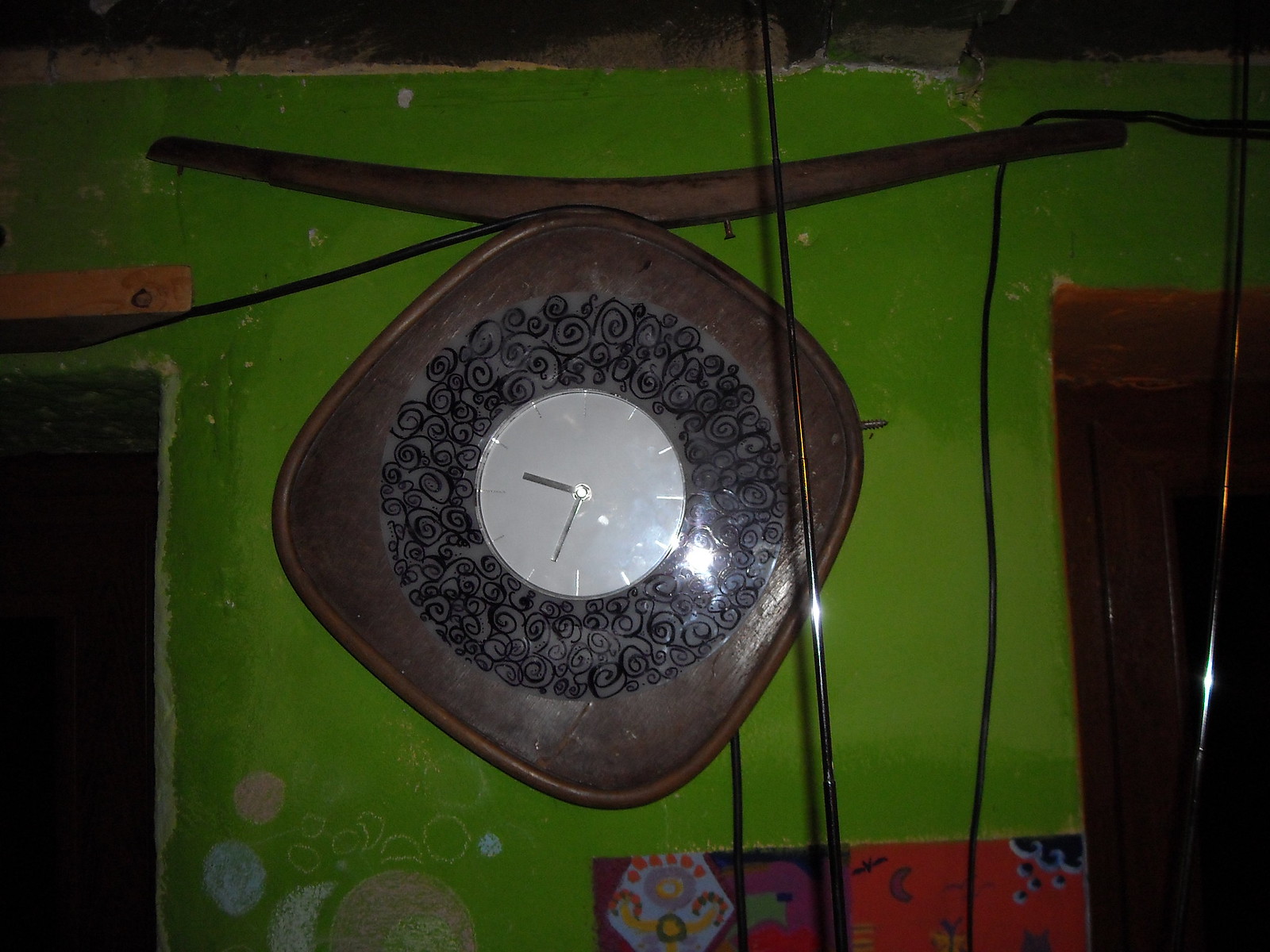The image features an antique, wall-mounted analog clock with a unique design. The clock has a brown, diamond-shaped wooden frame that is mounted with its tips at the top, bottom, left, and right, though the corners are curved rather than sharp. Notably, there is a visible screw on the right corner of the frame. The center of the clock consists of a grey circle adorned with black, lace-like designs encircling the white clock face. The clock face itself is circular, featuring silver dashed lines instead of numbers, and silver hands— a shorter one for the hour and a longer one for the minutes. The hour hand points between 5 and 6, while the minute hand is positioned between 9 and 10. Above the clock, there is a boomerang-shaped wooden ornament, also brown and made of wood. The background wall is painted a dark, bright green hue. Additional details include a wooden door located at the bottom right of the image, a second door on the left, and several black cables running across various parts of the scene, including above, behind, and below the clock. Other colors such as red, grey, white, and orange are visible at the bottom of the clock, adding to the intricate background details.